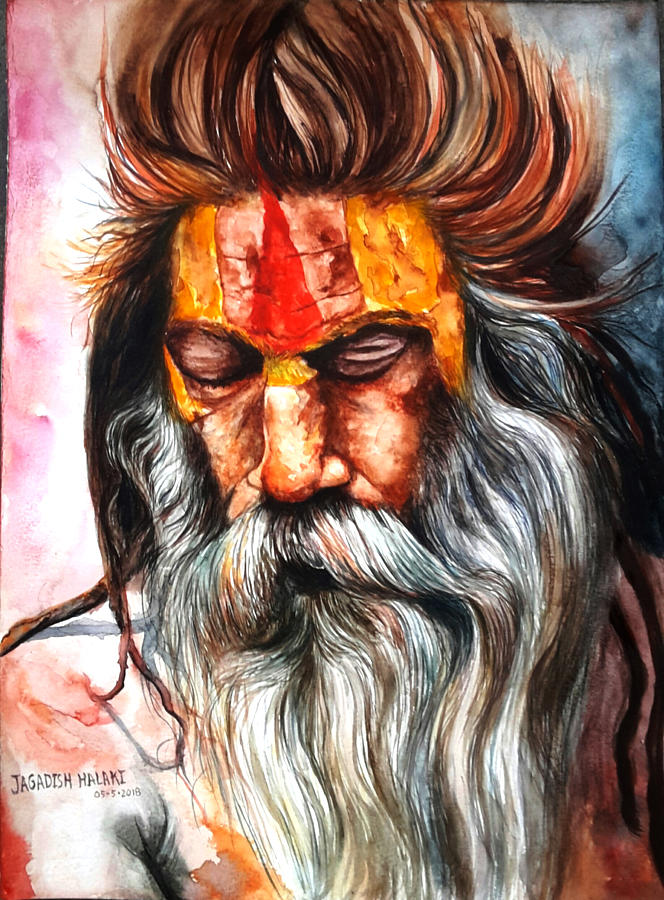This striking modern painting by artist Jagadish Halaki, signed and dated May 5th, 2018, depicts an older, rugged, and possibly indigenous or Indian man who resembles a lion. The man's auburn brown hair is styled in a tall, brushed-up manner, reminiscent of a rockabilly look, cascading down to his shoulders. His long beard and mustache are predominantly gray with some brown and tan streaks. His face is adorned with distinctive paint: a thin red triangle on his forehead, golden yellow paint along his temples extending down to his cheeks, and some white paint or mud on his shoulder. The man's eyes are closed, and he appears to be looking downward, adding to his contemplative and powerful demeanor. The background features a mix of muted reds, light pinks, light blues, and darker grays, with distinct and vivid strokes that suggest an oil painting technique. The overall composition is vivid and evocative, emphasizing both the man's majestic and weathered appearance.